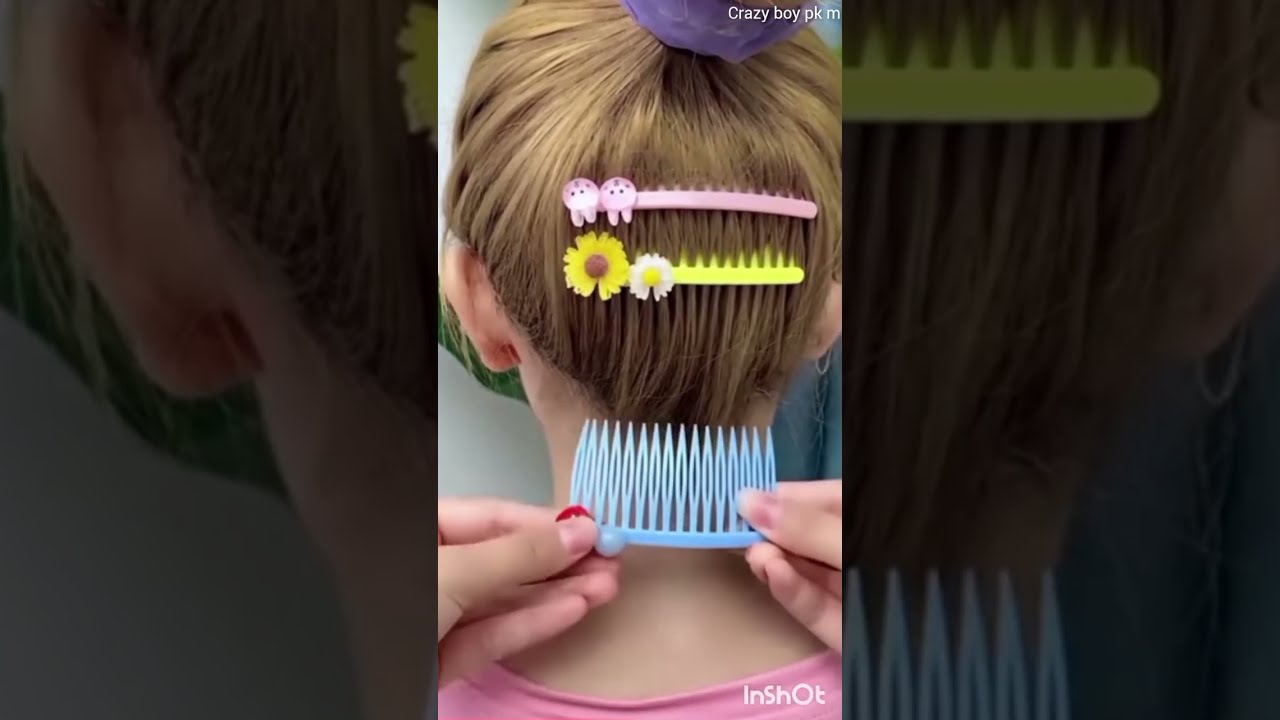The central image captures the back of a young girl or woman's head, her brown hair neatly swept into a ponytail or bun secured with a purple hair tie. Adorning her hair are a pink hair clip, embellished with small creature-like figures, and a yellow hair clip featuring flower symbols. Two hands can be seen near her neck, carefully positioning a blue comb-like hair piece into her hair, suggesting that her hair is being styled. The text "Crazy Boy PKM" is prominently displayed in the top right corner, while "In Shot" appears in the bottom right. Surrounding the central image, the background is filled with a darkened and zoomed-in version of the same picture, emphasizing the meticulous process of hair styling.